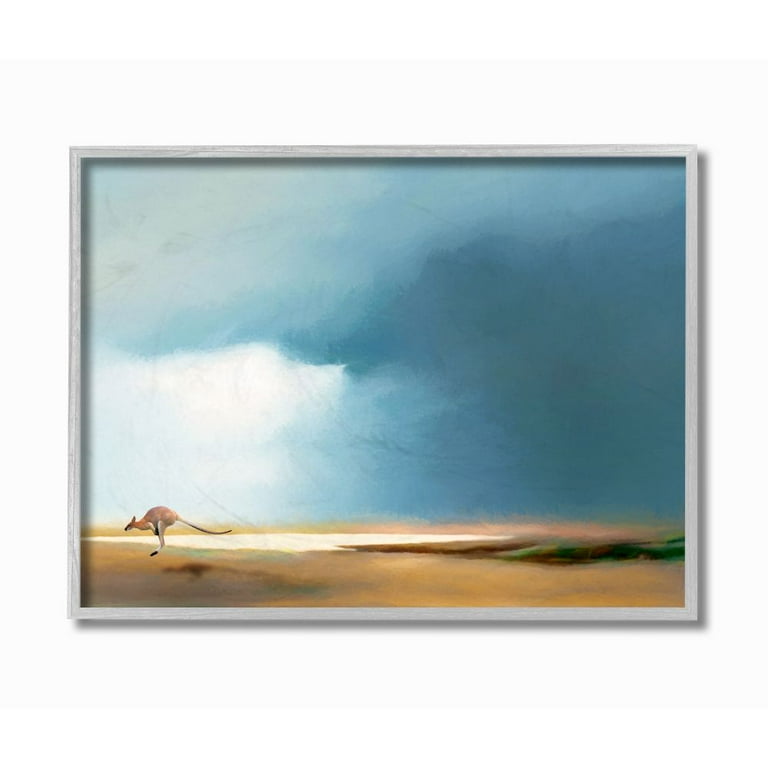The framed painting features a dynamic scene of a kangaroo mid-bounce across a desolate, sandy desert landscape. Positioned near the lower left corner, the kangaroo, with its bent head pointed toward the left edge and tail extending towards the painting's center, appears in midair with its legs straight beneath it. A clear shadow trails slightly behind and to the right of the animal. The thin gray or white-gray wooden frame surrounds the image, with light casting a shadow to the right and underside of it. The horizon line sits low, about 20% up from the bottom, featuring a sandy, tan foreground. A narrow white strip, potentially reflecting clouds, cuts across the landscape, punctuating the otherwise earthy tones. Above, the sky transitions from light, where the sun peers through white clouds on the left, to darker shades of blue and gray, hinting at a storm on the right. The overall ambiance suggests a stormy, yet intricate, portrayal of nature.